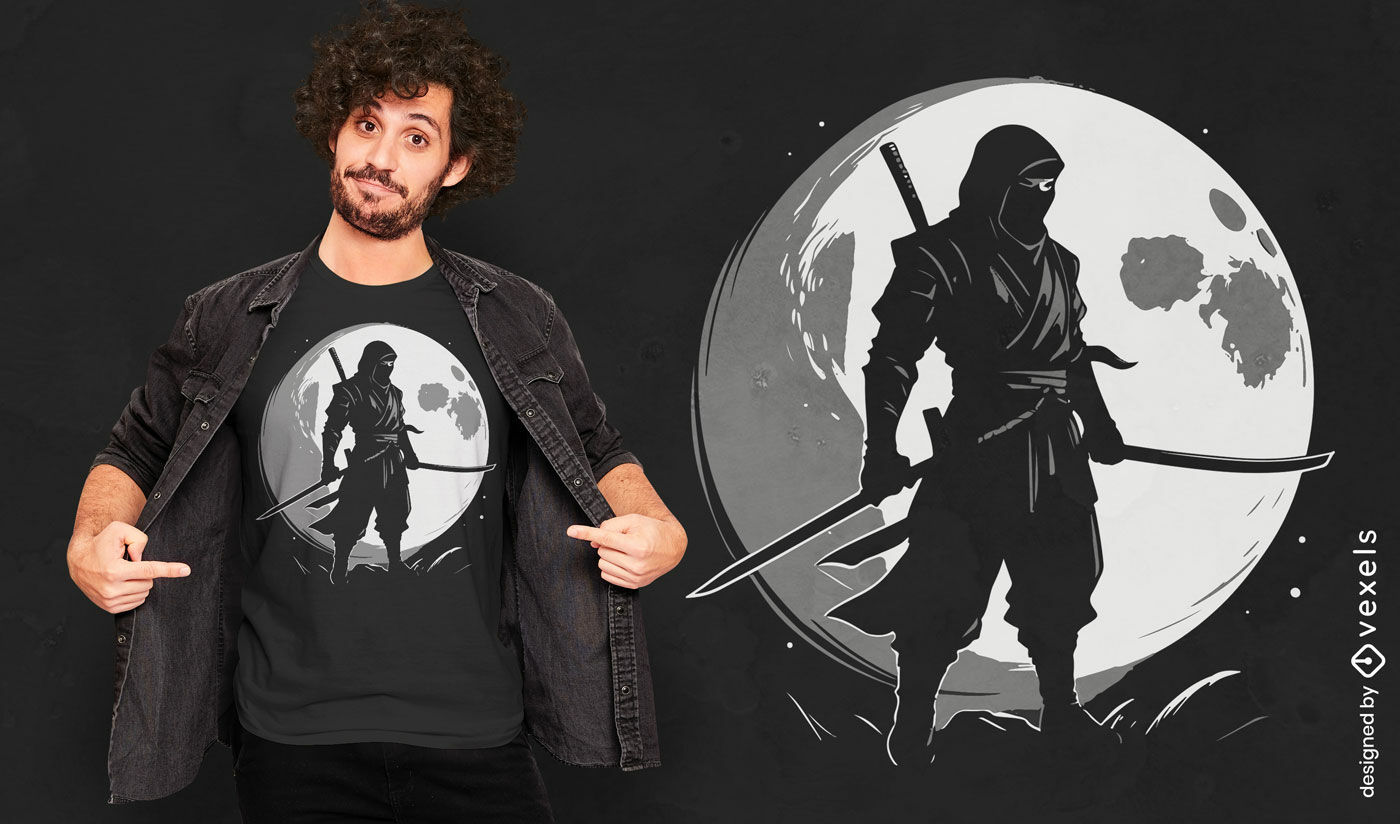The photograph features a man with bushy, curly black hair and a scruffy beard and mustache. He is dressed in a black denim jacket, worn open over a black t-shirt, and black jeans. The graphic on his t-shirt depicts a ninja warrior dressed in black, with a hood covering his head and only his eyes visible. The ninja is armed with swords in both hands, a sword at his belt, and another sword handle protruding from the top of his back. He stands on what appears to be rocks, with a white and gray globe, possibly the Earth or a moon, in the background. To the right of the man, the same ninja graphic from his shirt is displayed against a black background, zoomed in for better visibility. Vertical text on the lower right-hand corner reads "designed by Vexels."